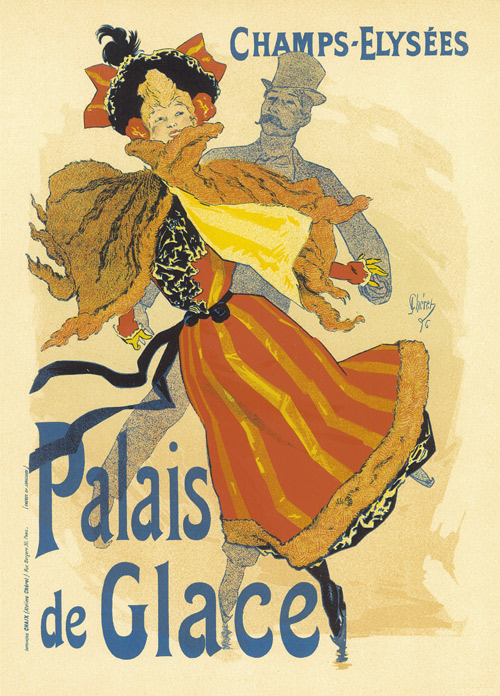This vintage poster, reminiscent of the art style of Toulouse-Lautrec, features promotional text in blue that reads "Champs-Élysées" at the top and "Palais des Glaces" at the bottom, with a signature dated '96. Dominating the scene is a vibrant woman in a red dress with golden yellow stripes, adorned with black lace at the bodice and a tight blue belt around her waist, typical of the late 19th century fashion. She wears a fancy feathered hat with red and yellow decorations, black heels, and a short, golden-colored cape draped over her shoulders. Her blonde hair and bright, happy demeanor make her the focal point of the composition. Nearly silhouetted behind her is a man with a top hat and black mustache, seemingly translucent with a blue hue, who appears to be her dance partner. This evocative image captures the lively and elegant spirit of the period, highlighting the allure of the famed Champs-Élysées and its attractions.